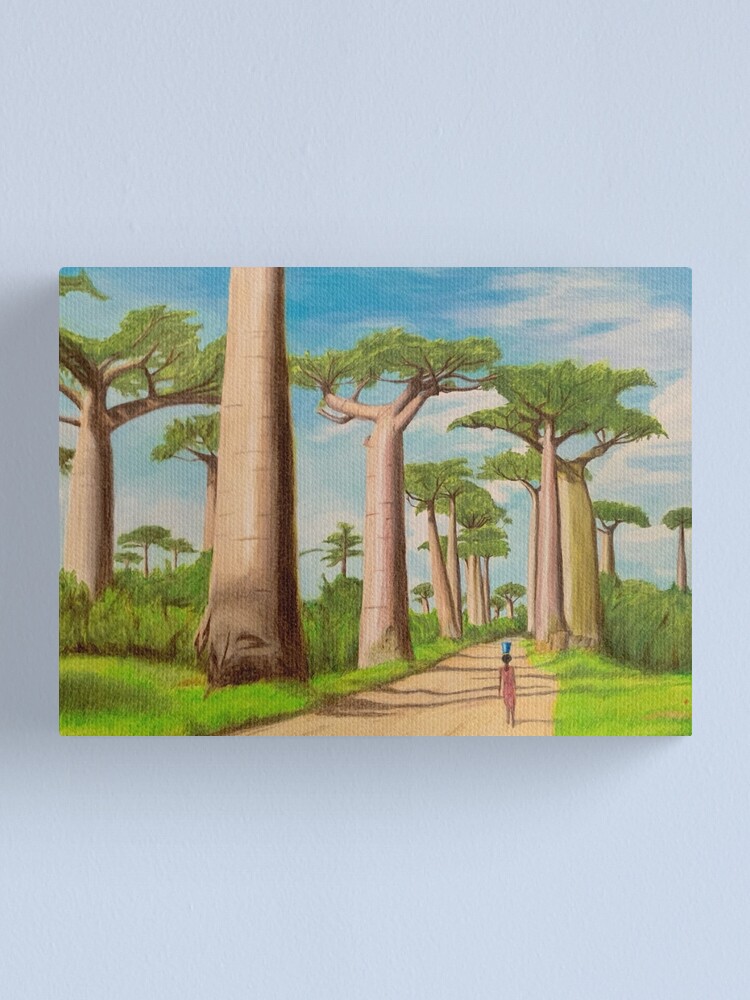This painting, an acrylic piece on canvas, depicts a serene scene of a woman walking down a beige dirt path that winds into the horizon, bordered by green grass and bushes. The woman, small in the bottom right corner of the painting, wears a pinkish-red dress and her black hair is tied back in a ponytail. She balances a blue bucket on her head as she strides along the path. Towering on either side of the path are distinctive trees characteristic of those seen in Africa off the coast of Yemen. These trees have smooth, thick, cylindrical trunks that ascend with no branches until they reach the very top, where they branch out into a Y shape with thinner branches and leaves. The sky above is a vibrant blue, adorned with wispy white clouds, enhancing the tranquil atmosphere of the scene. The painting is set against a light blue background, giving the impression that it is hanging on a blue wall.